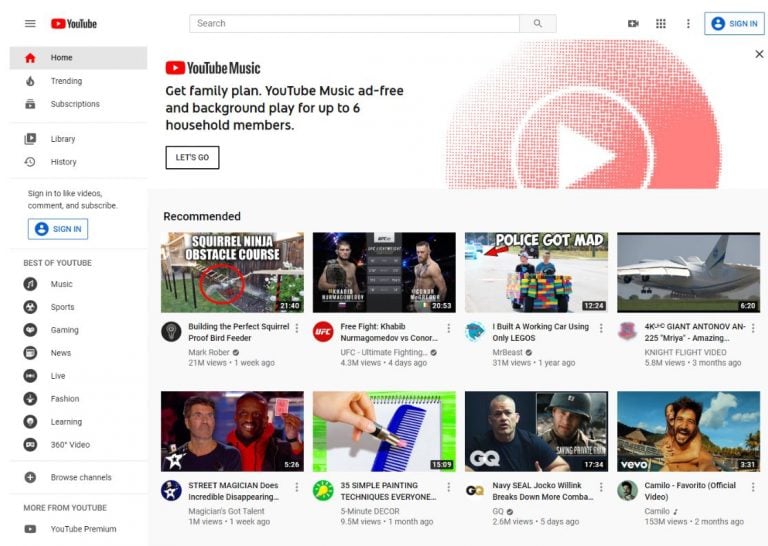This detailed caption succinctly captures the contents of the image described:

"Screenshot of a YouTube homepage taken on a computer. The YouTube icon is prominently displayed in the top left corner. The left-hand column features navigation options with icons and text, including a red home icon labeled 'Home,' followed by 'Trending,' 'Subscriptions,' 'Library,' 'History,' 'Sign in to like videos, comment, and subscribe,' with a 'Sign in' button. Below this, 'Best of YouTube' showcases categories like 'Music,' 'Sports,' 'Gaming,' 'News,' 'Live,' 'Fashion,' 'Learning,' and '360° Video.' Options to 'Browse channels' and 'More from YouTube' are also visible, with a 'YouTube Premium' button at the bottom.

In the central part of the screen, a YouTube Music advertisement banner at the top announces, 'Get Family Plan, YouTube Music ad-free and background play for up to six household members,' featuring a large red and white play button prominently.

Below the advertisement are two rows of recommended videos. The eight different video thumbnails displayed are titled: 'Building the Perfect Squirrel Proof Bird Feeder,' 'Free Fight' showing a fighting match, 'Lego Car,' 'Plane,' followed by 'Street Musician,' 'Painting Techniques,' 'Navy SEAL,' and a user-uploaded video."

This descriptive caption effectively conveys the layout and content of the YouTube homepage displayed in the screenshot.